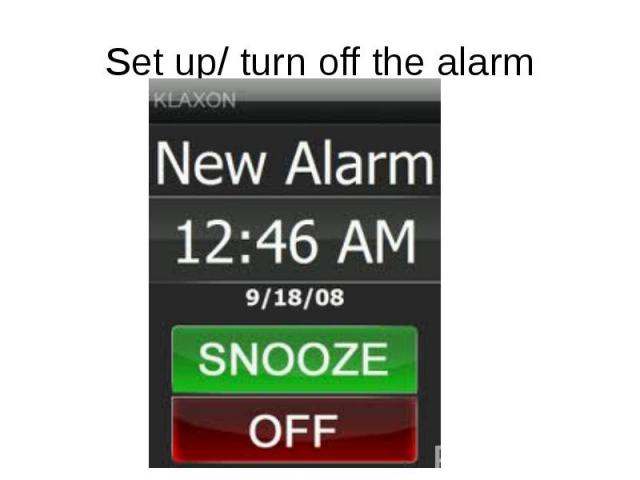The image displays a digital alarm clock interface with various elements and indicators. At the very top of the screen, the text reads "Set Up / Turn Off the Alarm." Directly below this header, there is a section with a dark gray background featuring the word "KLAXON" in all capital letters, followed by "New Alarm" in white font.

In the upper left-hand corner, "1246 AM" is displayed, with the date "9/18/08" below it, indicating September 18, 2008. Both the time and date are separated by horizontal lines. The middle part of the image showcases these details prominently.

Towards the bottom of the interface are two rectangular buttons of the same size. The first button is green with the word "SNOOZE" written in all capital letters in white font. Below it, there is an identical red rectangular button with the word "OFF" also in white uppercase letters.

The background colors throughout the interface are a mix of black, white, and shades of gray, enhancing the contrast and making the text stand out. Overall, the setting appears to be an alarm setup screen, likely used in a home environment to manage wake-up alarms.